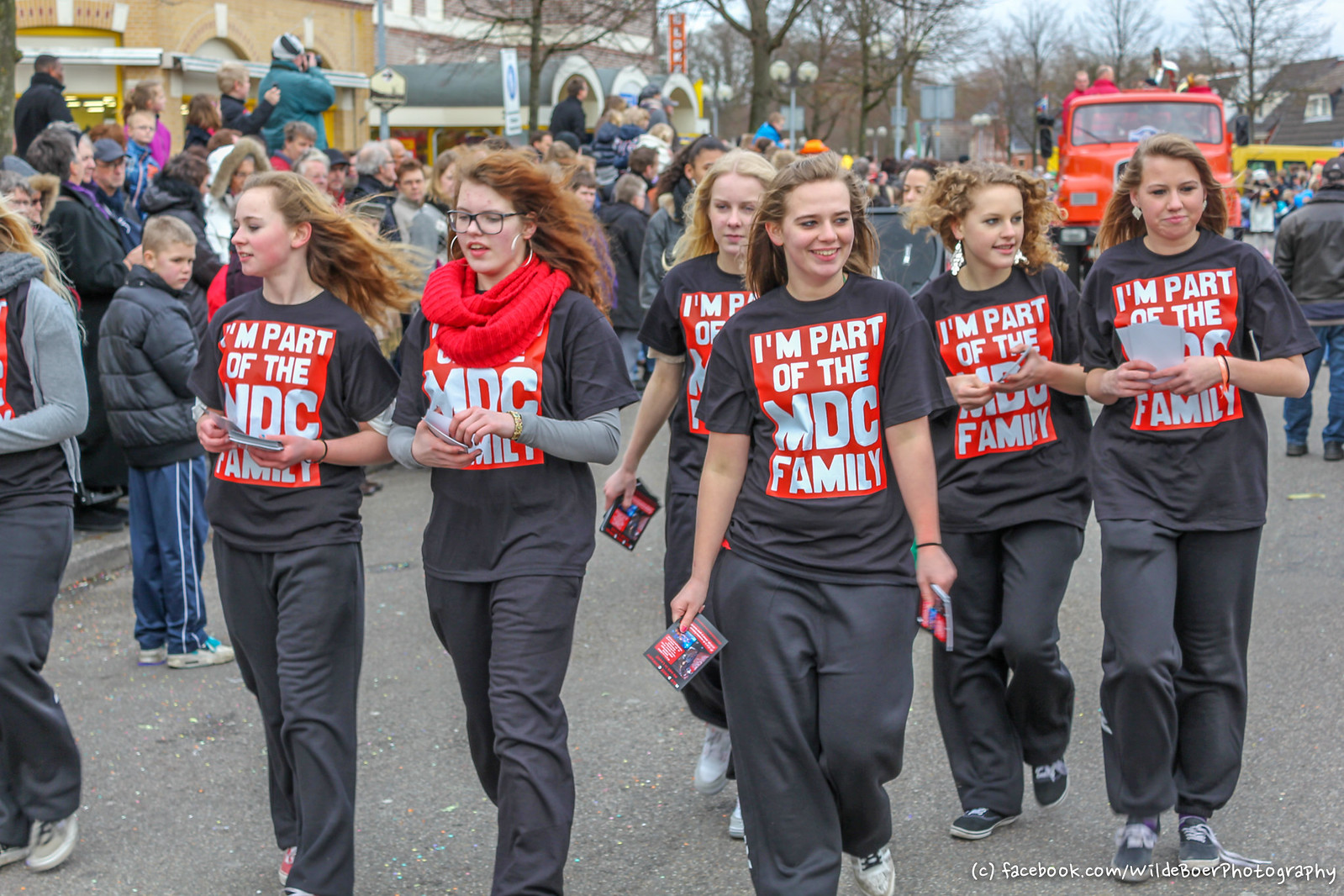The image is a vibrant full-color photograph capturing an outdoor parade or march, likely in the fall as indicated by the leafless trees in the background. The focal point is a group of seven young women walking towards the camera, centrally aligned. They are all dressed identically, wearing black t-shirts with a large red rectangle on the front that reads, "I’m part of the MDC family," paired with black pants and dark-colored tennis shoes. One of the girls is notably wearing glasses. They each hold small cards or flyers in their hands. Surrounding them, a large crowd fills the sides of the street, dressed warmly in winter coats, suggesting cooler weather. In the distance, on the right side, there is a red truck and a yellow school bus, partially visible amidst the throng of spectators. The bottom right corner of the photograph contains a watermark: "facebook.com/wildboarphotography."